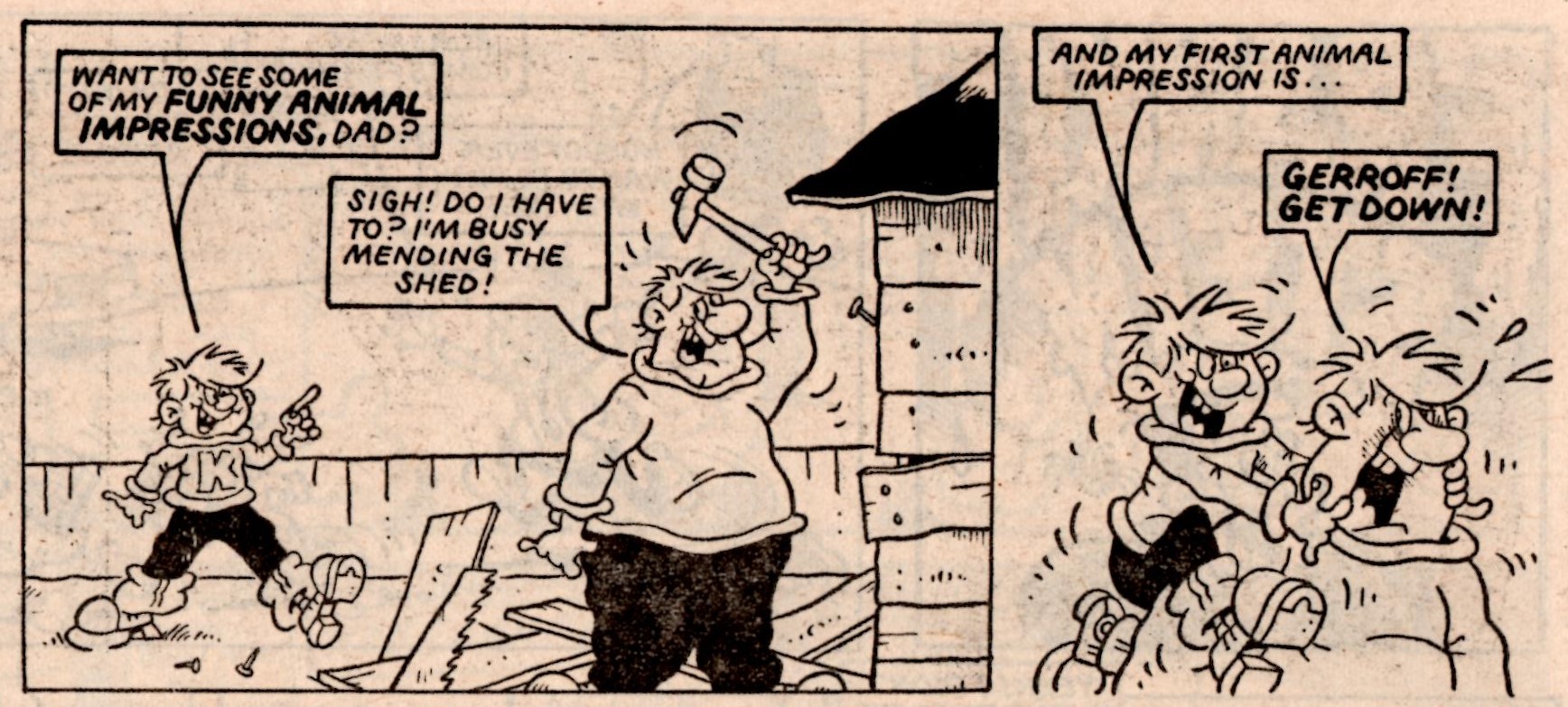This black-and-white comic strip, with a landscape orientation, is reminiscent of the Sunday funnies and consists of two panels. In the first panel, which takes up two-thirds of the strip, a father is seen mending a shed with a hammer raised near a nail on a building. Scattered around are a saw and some wooden boards. The father, clad in black pants and a white shirt, looks weary as he responds to his son who is eagerly approaching him with the question, "Want to see some of my funny animal impressions, Dad?" The father's speech bubble reads, "Sigh, do I have to? I'm busy mending the shed." A simple fence forms the backdrop of this scene, beneath a blank sky. In the second, smaller panel, the son, also dressed in black pants and a white shirt, has leaped onto his father's shoulders, clasping his face from behind. As he announces his first animal impression, "And my first animal impression is...," the father groans in pain, his speech bubble exclaiming, "Groff, get down!"